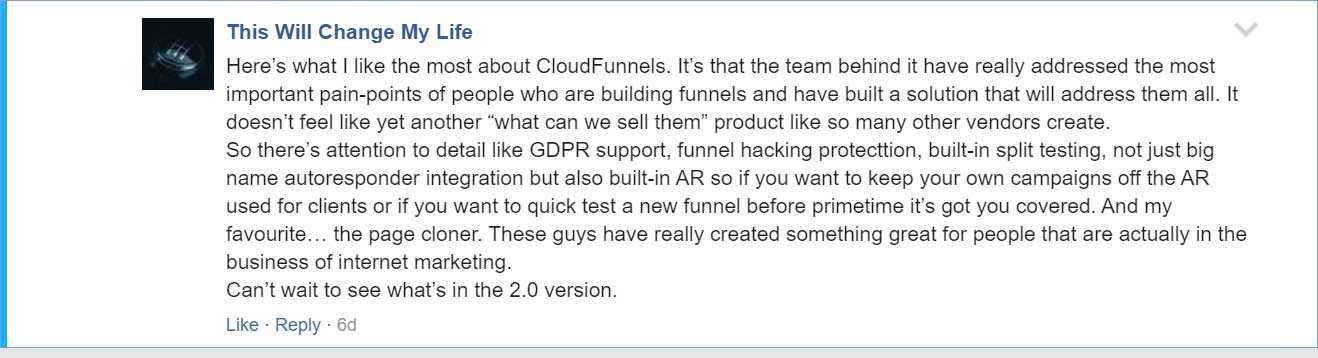Here's a cleaned-up and detailed caption for the described image:

---

**Title: This Will Change My Life**

In this post, the user praises the Cloud Funnels platform for its comprehensive features designed to address the primary pain points of funnel builders. Highlighted attributes include GDPR support, built-in funnel hacking protection, and split testing capabilities. Not only does Cloud Funnels integrate smoothly with major autoresponders, but it also offers a built-in autoresponder (AR). This flexibility allows users to keep their campaigns separate from clients' or to quickly test new funnels before a major launch. The user particularly appreciates the page cloner feature, emphasizing that the developers have created a genuinely effective tool for internet marketers. They eagerly anticipate what enhancements version 2.0 will bring.

---